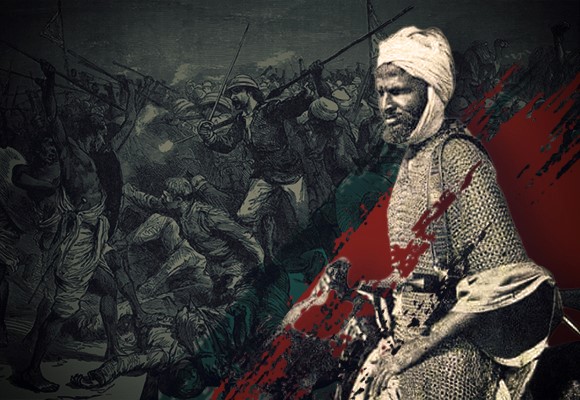This detailed, hand-drawn or AI-sourced image depicts an ancient war scene with a stark black and white background, punctuated by splotches of red and a line of blue shading in the middle. At the forefront, a bearded Middle Eastern man, recognizable by his distinctive head garb—a white cloth wrapped under his chin and around his head—stands facing left, revealing his injured left hand and different sleeves on his attire. He is clad in soldier gear with metal squares on top, straps descending to his waist, and is engaged in combat amidst a chaotic melee. The scene features a mix of European and tribal combatants, some wielding spears and swords in intense hand-to-hand fighting. On the right side, near a patch of red, an individual in chain mail and a full headdress stands, adding to the historic and diverse nature of the battle depicted.